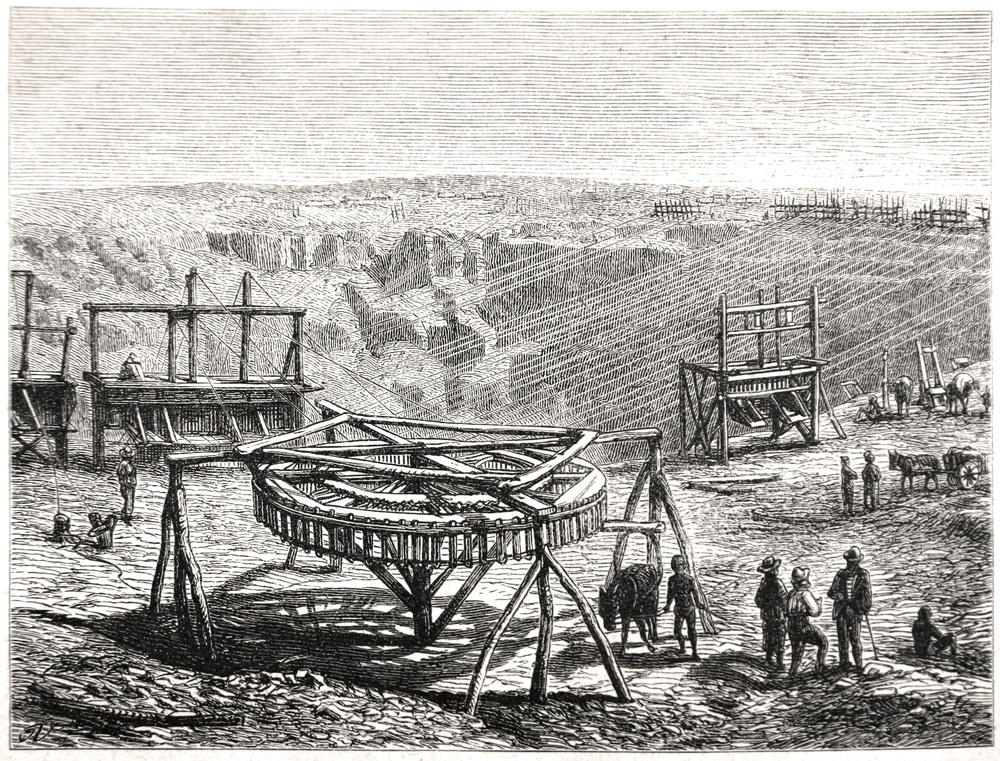The image is a highly detailed black and white sketch, possibly created using pencil or charcoal, resembling an old etching or art print depicting a bustling construction scene. In the foreground on the bottom right, there are three individuals standing together, and a fourth person is seated on the ground next to them. The main feature of the scene is a large wooden contraption with a horizontally oriented wheel mounted on a post. A horse or donkey is attached to spokes coming out of the wheel, seemingly involved in turning it, guided by a person standing next to the animal.

Surrounding this contraption are other wooden structures with platforms, elevated from the ground, indicating an active work site. The backdrop lacks trees, suggesting a flatland, possibly a large crater or dirt-filled area with fences in the distance. The sky is represented by white space with black lines. Various people and animals populate the scene, contributing to the sense of bustling activity typical of a dynamic construction site.